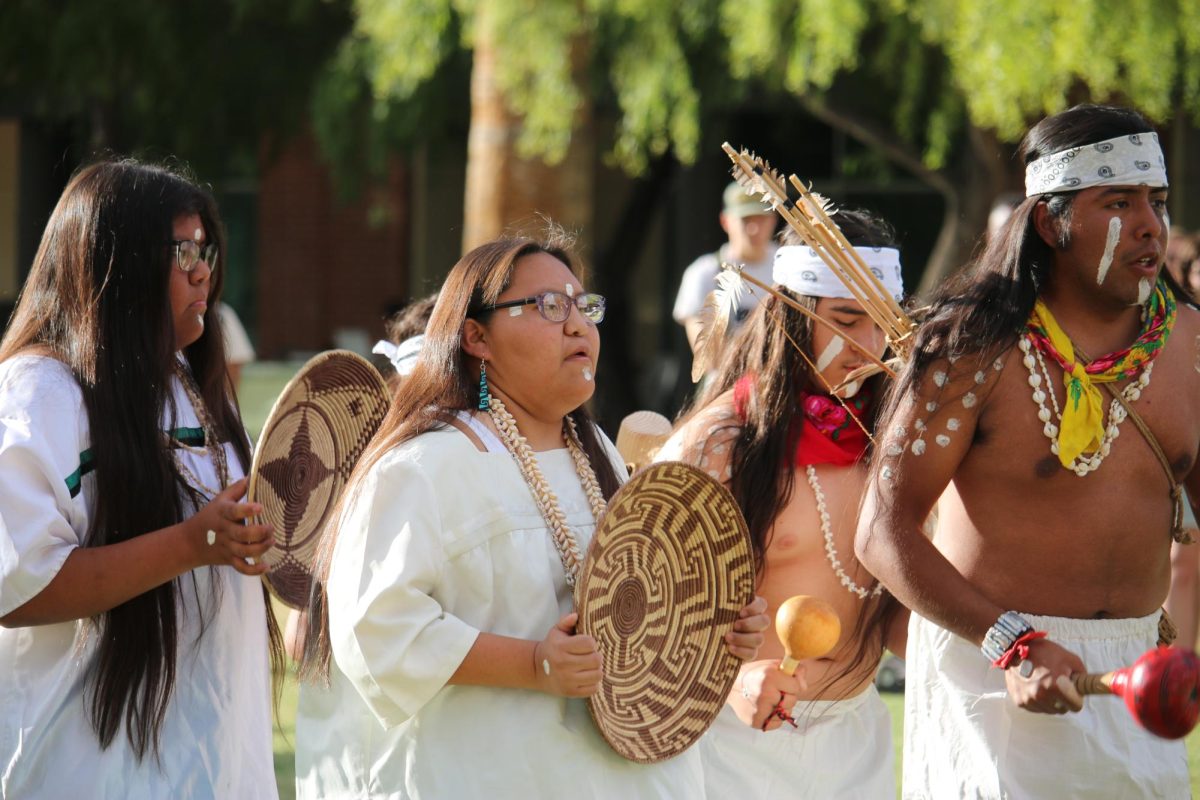The image captures a Native American event, likely a powwow, set in an outdoor public area with trees and a building in the background. In the foreground, four individuals stand out in traditional attire: two shirtless men on the right and two women on the left. 

The first man, positioned at the front on the right, wears a white and black headband, a seashell necklace, and white face paint beneath his eyes and lips, along with white dots on his shoulder. He carries a red gourd rattle and has a bow with arrows slung over his back. Behind him stands another shirtless man, adorned similarly but with a red bandana around his neck and a yellowish gourd rattle.

To the left of the men, a woman dressed in a white robe holds a woven basket adorned with tribal shapes. She wears glasses, a similar seashell necklace, and face paint like the men. Next to her stands a younger woman in a white robe featuring a green stripe across the chest, holding a darker star-patterned woven bowl. Both women have long dark hair. In the background, some onlookers and a man wearing a hat can be seen. The event exudes a vibrant cultural atmosphere, enriched by the participants' intricate traditional outfits and shared activities.